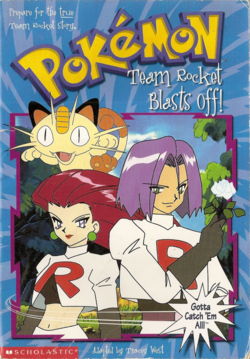The image is a colorful book cover of a Pokémon comic. The background is predominantly blue with streaks of gray. In the upper left corner, there's small text that appears to read, "Prepare for the true team... stay Team Rocket, stay." Below this is the large, yellow title "Pokémon," outlined in purple, with an accent over the "é" to emphasize the pronunciation. Beneath the title, white thin letters spell out "Team Rocket Blast Off."

The main illustration shows three figures. To the top left, a cat-like creature with a horn-like protrusion on its head stares wide-eyed at the viewer. Below the creature, a woman with bright red hair wears a white shirt emblazoned with a large red "R." Next to her, on the right, is a man with shoulder-length gray hair, also wearing a white shirt with a red "R." The man has gray gloves and is holding a white flower in his bent arm. Both characters have an action figure-like appearance. 

In the lower right corner, a white starburst contains the phrase, "Gotta catch 'em all," and in the lower left corner, a red bar with the word "Scholastic" in white confirms this as a book cover.